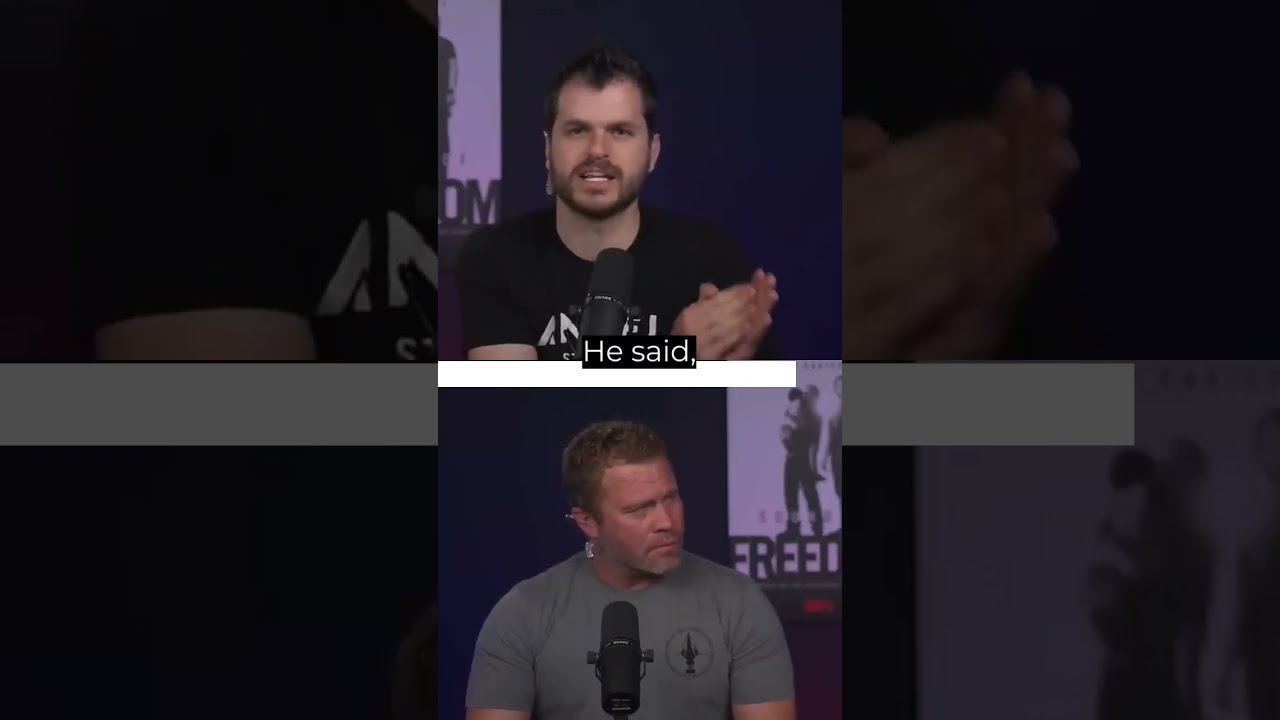The image is a wide rectangular composition, predominantly showcasing a central tall rectangular section that appears to be a screenshot of a video chat or a show. This primary section displays two white men speaking to a camera, positioned one above the other, set against a purple backdrop with a purple and black poster partially visible behind them. The man at the top, who has paler skin and brown hair, is dressed in a black t-shirt with white writing and speaks into a microphone. The term "Freed" is partially visible in the background, hinting at a movie or TV show title. The man on the bottom, wearing a gray shirt and having blonde hair, also speaks into a microphone and looks to his right. 

Flanking this central image on both the left and right are even taller, wider sections that are darker, close-up zooms of the central image, creating a blurry and shadowed effect. This creates a mirrored effect that emphasizes the central image's content. The background and setting suggest that these men are part of a panel or a Q&A session, as implied by the shared purple theme and the continuity of the poster featuring the partially readable words "Freed," "O," and "M." The shared colors across the image include various shades of purple, black, white, and gray, creating a cohesive yet dynamic visual narrative.